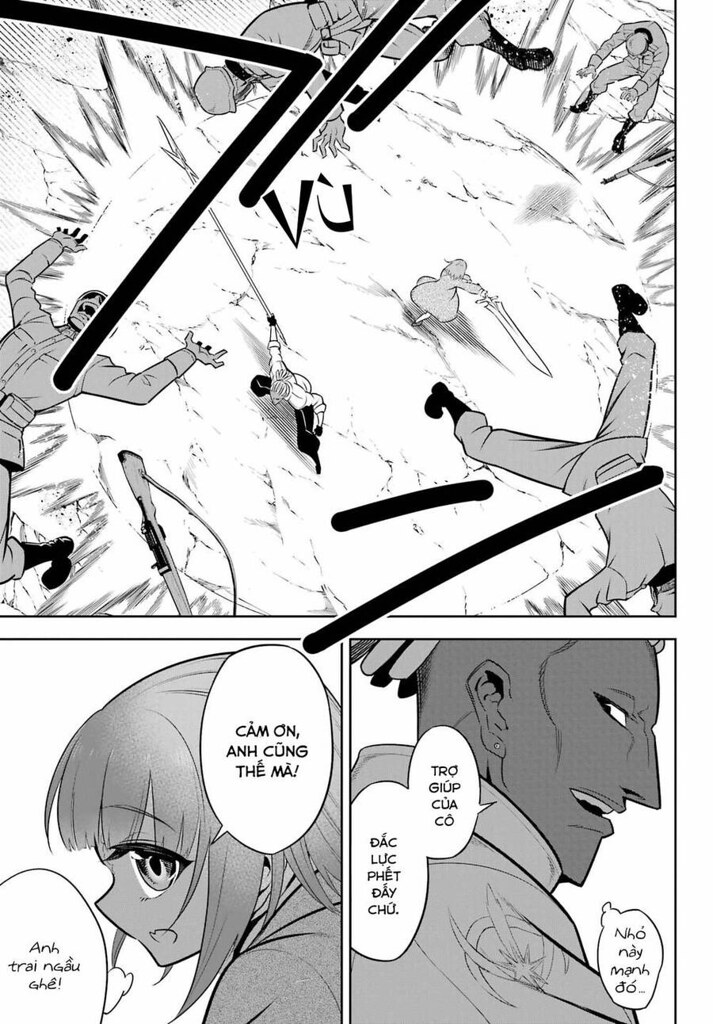The black and white image resembles a page from a manga or anime-style graphic novel, divided into three distinct scenes. The top panel captures a dynamic combat scene, where a girl wielding a sword and a man with a spear fend off multiple attackers. The fray unfolds with the attackers, who appear to be soldiers, being forcefully flung away, one even losing grip of a rifle. The aggressors have been rendered visually defeated, scattered across the panel.

In the bottom left panel, the girl from the fight appears slightly turned to the side, expressing something in what seems to be Vietnamese, captured in a speech bubble and a thought bubble. Her expression adds a dramatic flair to her words. The bottom right panel shows a man, potentially one of their opponents from the fight, with distinct angular features and a menacing expression. He also speaks in the same foreign language, with his dialogue presented in speech and thought bubbles, adding to the narrative's intrigue. The entire artwork is executed in shades of black, gray, and white, emphasizing the intense and dramatic nature of the scenes.